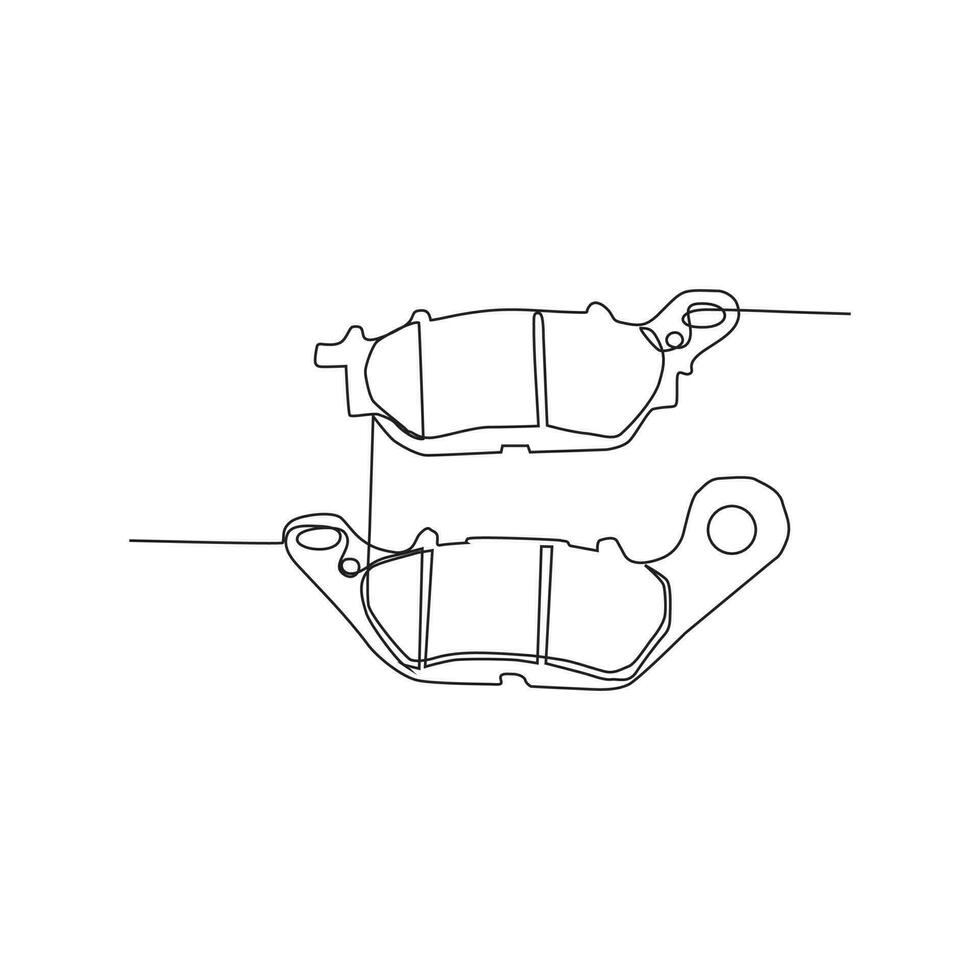The image showcases a simple black ink line drawing on a white background, resembling either a schematic diagram or a track design. Dominating the image are two elongated ovals with detailed black outlines. The top right of the upper oval features an extension with a hole, through which a string or wire loops and extends rightward. This string continues to the next object below, creating a sense of connection between the two. The lower object, nearly identical to the upper one, also has extensions but with noticeably larger knobs on its sides. Both objects appear to be part of a contraption or device, with intricate connections and pathways depicted by the looping wires, offering a technical yet artistic representation of their design.